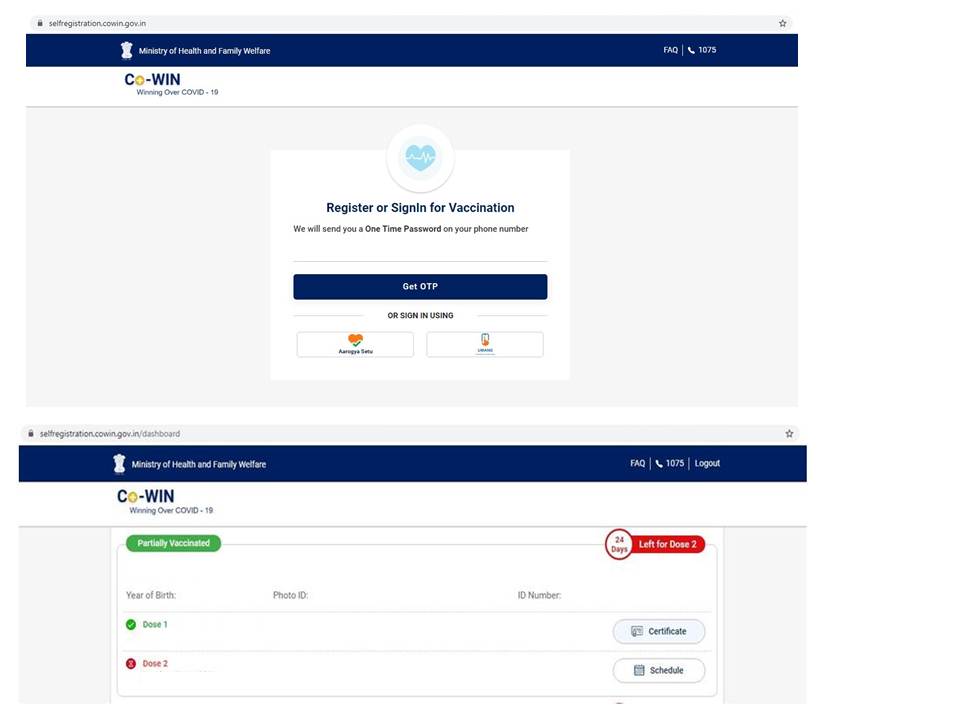This image, sourced from a website, features a prominent banner at the top indicating its affiliation with the Ministry of Health and Family Welfare. Beneath this header, bold text reads "Co-WIN" with the tagline "Winning over COVID-19". 

In the central portion of the page, a stylized heart with a heartbeat line, colored in light blue, captures the viewer’s attention. Within this graphical heart, the text prompts users to "Register or Sign In for Vaccination". Instructions follow, stating: "We will send you a one-time password on your phone number," accompanied by a faint green line and a button labeled "Get OTP". Below this, alternative sign-in methods are offered with two additional clickable boxes.

As you scroll down the page, it seemingly merges with another section of the website, again displaying the Ministry of Health and Family Welfare header. This lower section includes links to an FAQ section, a phone support section, and a logout option.

The recurring "Co-WIN: Winning over COVID-19" motif is again visible, accompanied by fields indicating "Partially Vaccinated". Users are prompted to input details such as year of birth, photo ID, ID number, and vaccination status, highlighting dose one and dose two, which are distinctly marked in red to signify the need for scheduling.